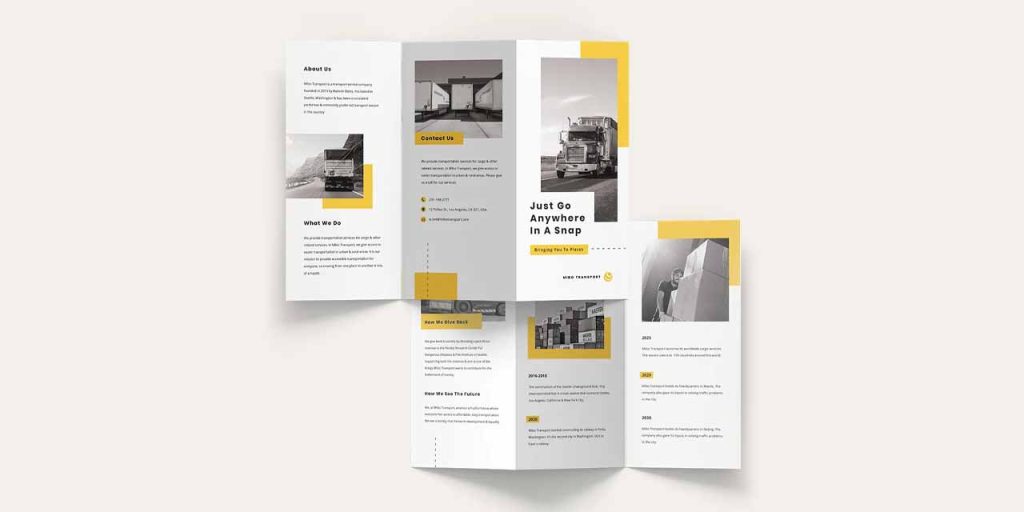The image depicts two open pamphlets laid out against a light beige-gray background. Both pamphlets, which have a white background, are tri-fold and have been unfolded to reveal their interior panels. The upper pamphlet, slightly overlapping the lower one and positioned more to the left, displays a clear arrangement of black-and-white images and text. Each panel of the pamphlets contains one image, bordered partially with yellow accents that highlight specific words and areas. On the top pamphlet, the cover features a semi-truck and the phrase "Just go anywhere in a snap," hinting at the service being offered. Inside, the pamphlet provides information with headers like "About Us" and "What We Do," accompanied by images depicting various aspects of truck-related activities. The lower pamphlet, although partly obscured, also follows a similar pattern with black-and-white photos, yellow highlights, and text that presumably details the steps involved in the trucking profession, including a picture of a person carrying multiple boxes. The overall presentation and repeated use of color suggest the pamphlets are marketing materials for a trucking company.